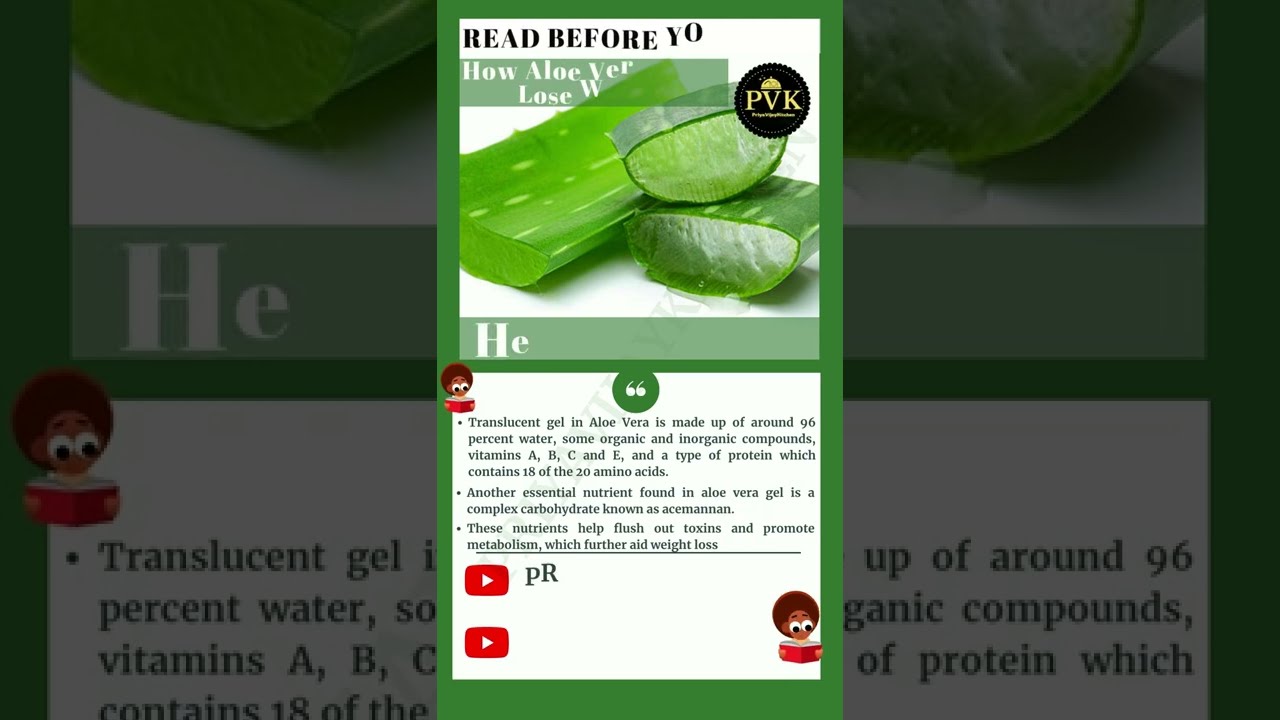The image is an informative graphic about aloe vera, featuring various elements and text. The background is predominantly green, and at the top of the image, there's a heading that reads "Read Before Yo: How Aloe Vera Lose W." Toward the center, white letters spell out "H E." In the upper right corner, there's a black circle with gold letters that read "PVK." The top section of the image includes a photo of an aloe vera leaf, sliced to reveal its smooth green core and translucent gel. Below this, the image contains multiple bullet points outlining the composition and benefits of aloe vera. The first bullet point mentions that the translucent gel of aloe vera is composed of around 96% water, along with various organic and inorganic compounds, vitamins A, B, C, and E, and a type of protein containing 18 of the 20 amino acids. The second bullet point highlights an essential nutrient found in aloe vera gel, a complex carbohydrate known as acemannan. The final bullet point explains how these nutrients help flush out toxins, boost metabolism, and aid in weight loss. Additionally, there are two YouTube icons at the bottom of the image.